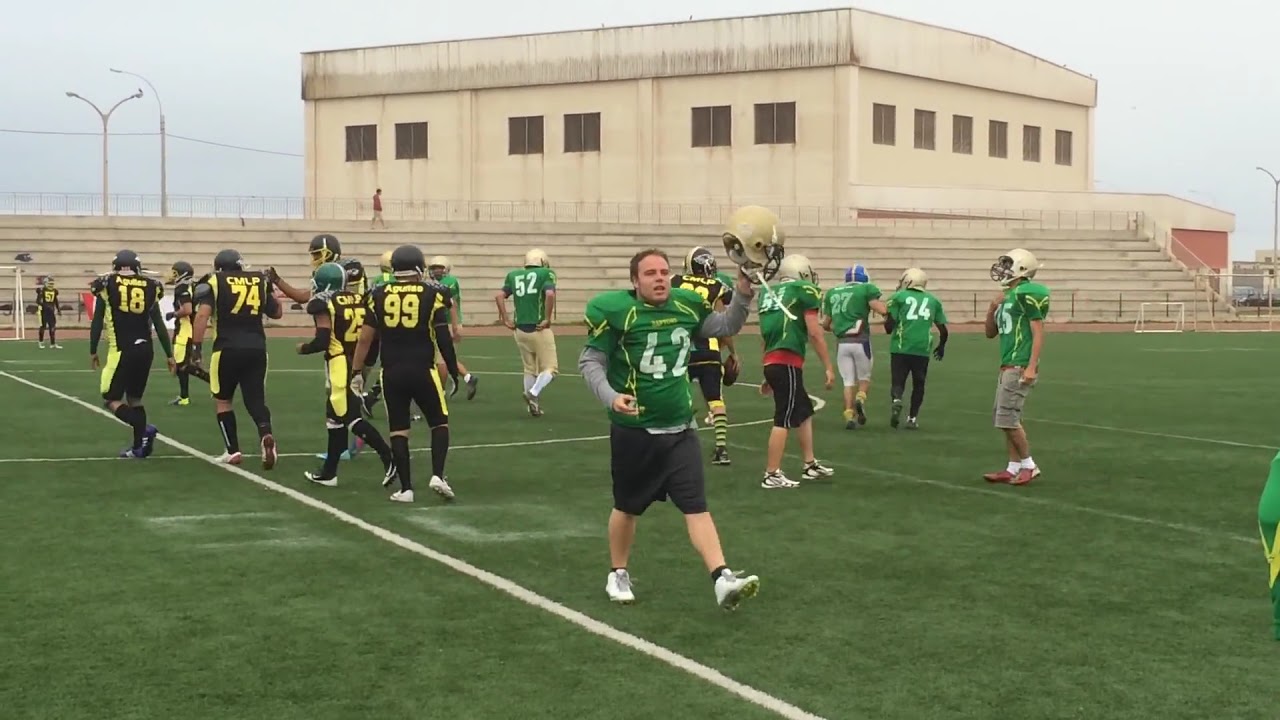The image captures an outdoor football game in action on a green grassy field, amidst a foggy, gray sky. In the background stands a large, three-story, yellow-tan building, partially obscured by tall, cement bleachers that rise up in at least eight rows. Streetlights can be seen beyond the bleachers, illuminating parts of the scene. On the field, two teams are distinguishable: one in green jerseys with gold helmets and another in black uniforms with yellow lettering, black helmets, and black shorts. Dominating the foreground is a Caucasian player wearing a green jersey with the number 42, dark shorts, white tennis shoes, and black socks. He is depicted lifting his helmet, as if waving someone down, drawing significant attention with his short hair and poised stance.